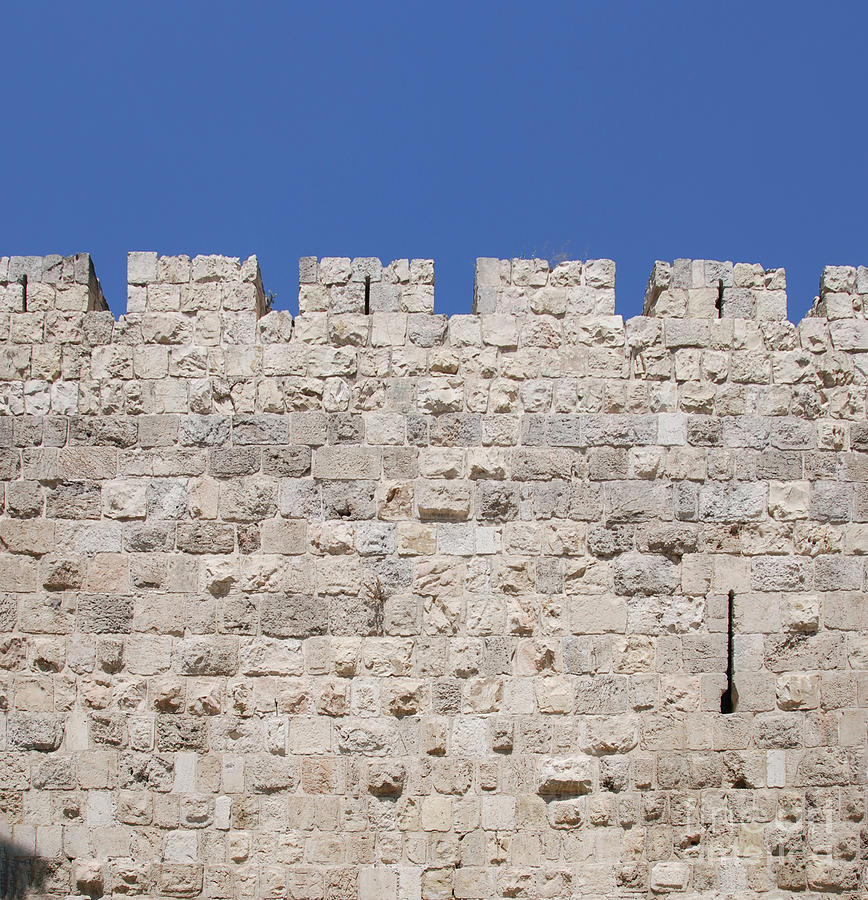The photograph captures the top portion of a well-preserved castle wall under a solid medium blue, cloudless daytime sky. The stone wall is constructed from tightly fitted light gray and off-white stones, giving it a textured, historical appearance. The wall features the iconic jagged and squared-off crenellations, designed to protect archers during medieval times. Additionally, there is a narrow vertical slit in the wall, likely a loophole for archers to shoot through while remaining shielded. The sun shines brightly, casting a clear, detailed view of the stonework and contributing to the vibrant contrast against the blue sky.